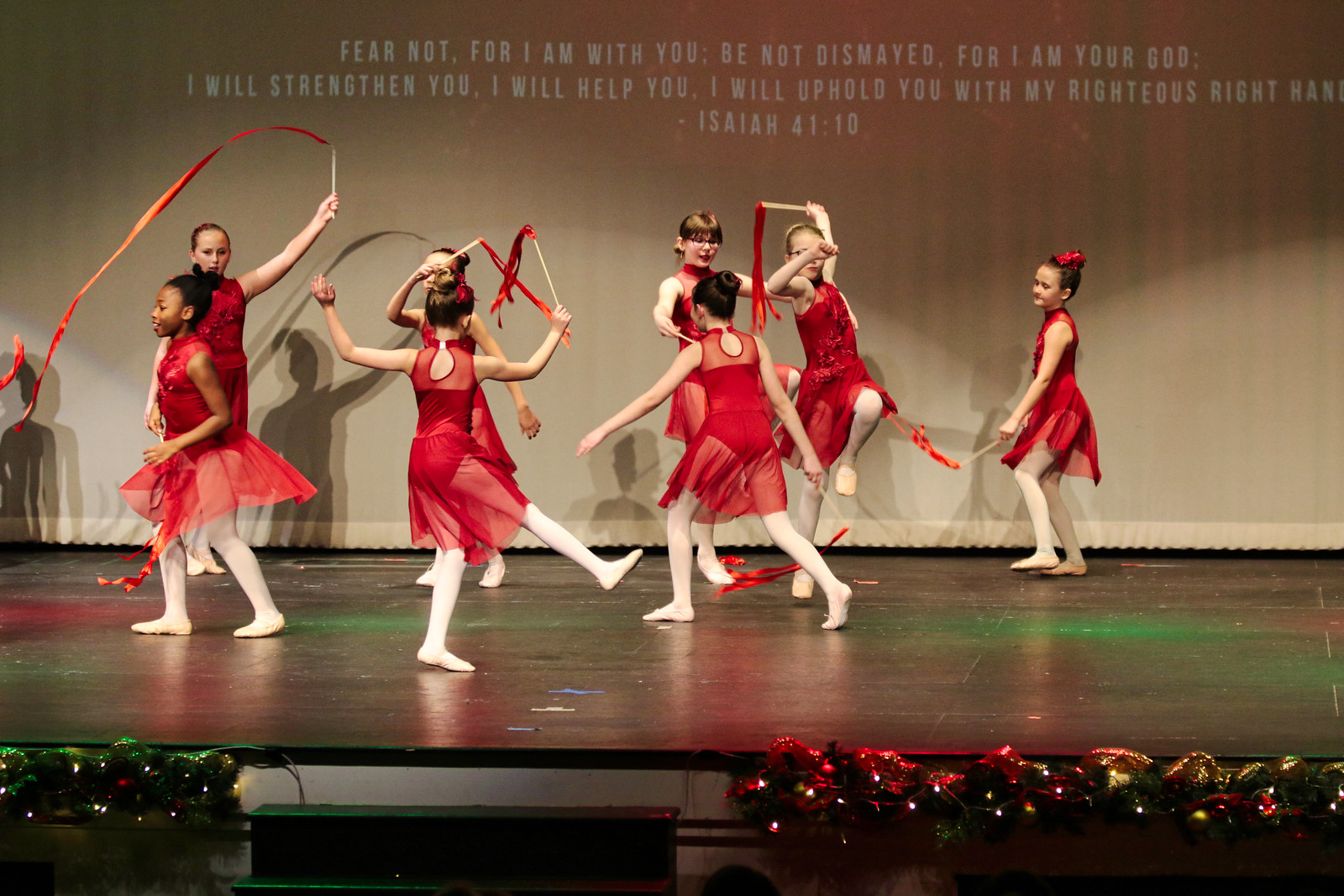The photograph captures a lively performance of young girls dancing on a stage, donned in red leotards with matching silk skirts and white tights. Each girl wields a stick adorned with flowing red ribbons, adding a dynamic visual element to their movements. The black wooden stage they dance on is adorned with shiny, crinkly decorations in red, gold, and green, enhancing its festive appearance. Behind them, a beige curtain serves as a backdrop, featuring a prominently displayed biblical quote: "FEAR NOT, FOR I AM WITH YOU; BE NOT DISMAYED, FOR I AM YOUR GOD; I WILL STRENGTHEN YOU, I WILL HELP YOU, I WILL UPHOLD YOU WITH MY RIGHTEOUS RIGHT HAND – ISAIAH 41:10." The stage's edge sparkles with decorative lights, creating an enchanting atmosphere for the heartfelt performance.